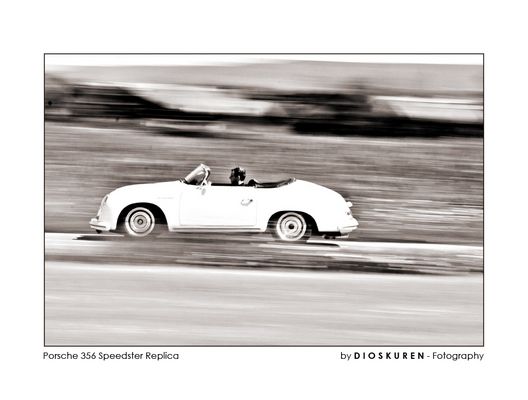In this black-and-white artistic photograph, a vintage white Porsche 356 Speedster Replica is caught in motion traveling towards the left, slightly off-center. The vehicle is depicted in profile with its top down, driven by a man. The high speed of the car is conveyed through the blurred foreground and background, creating streaks that emphasize its rapid movement. The background hints at the presence of a building, rendered indistinguishable due to the motion blur. The street the car is driving on appears white in the monochrome color palette. Framing the image is a thin black border, and captions are strategically placed at the bottom corners: "Porsche 356 Speedster Replica" on the left and "By Dioskurin Photography" on the right, the latter bolded and in all capital letters.